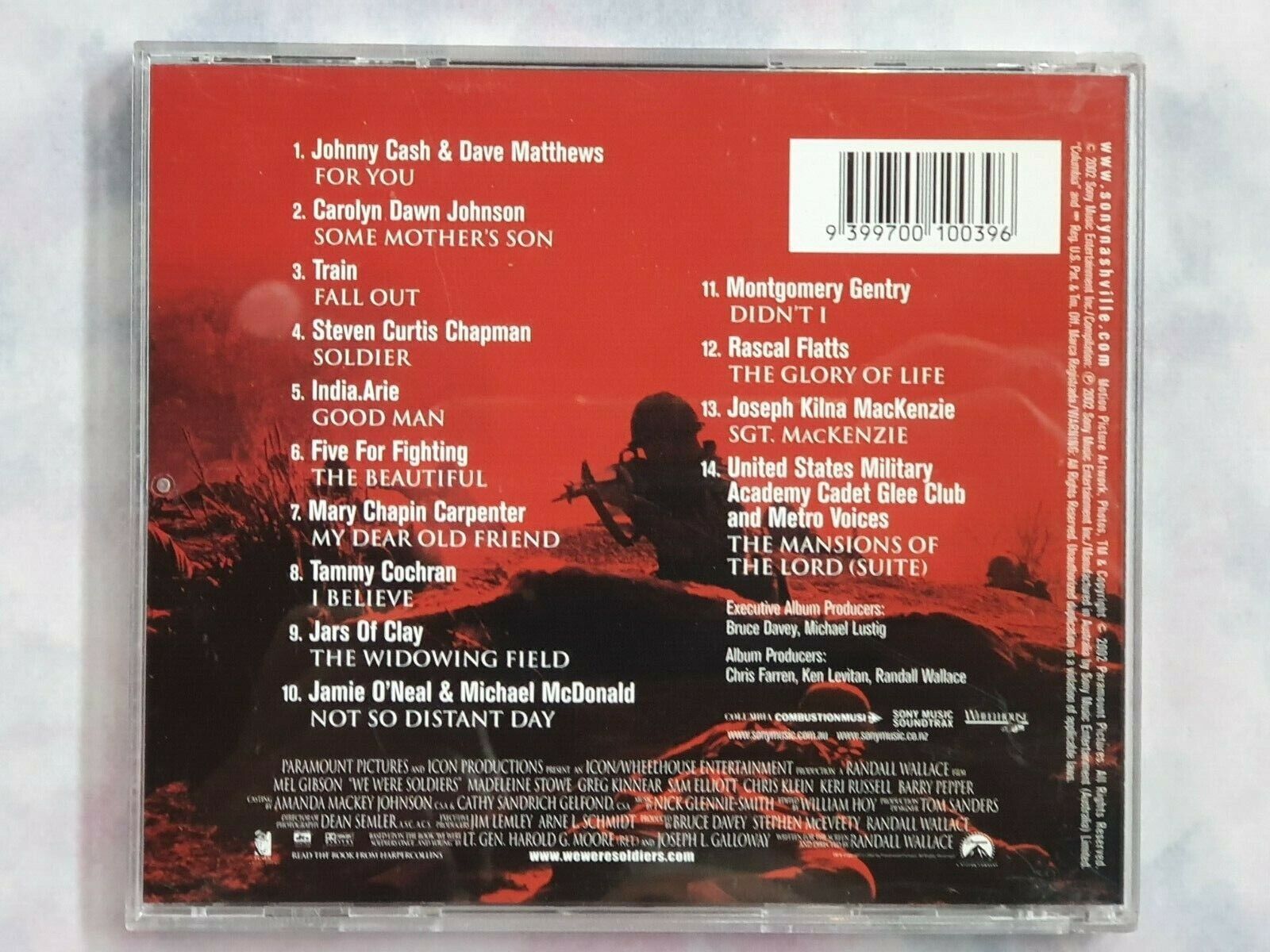This photograph features the back of a CD case set against a mottled gray background. The CD cover itself is red and prominently displays a silhouette of a soldier with a helmet and machine gun, with another figure lying down behind a small hill and vegetation elements like a bush and grass to the left. The CD serves as the soundtrack for the movie "We Were Soldiers" and includes 14 tracks listed in white text—10 on the left side and 4 on the right. The songs are by various artists, with standout tracks including "For You" by Johnny Cash and Dave Matthews, "Some Mother's Son" by Carolyn Dawn Johnson, and "Fallout" by Train. Other notable artists featured are Stephen Curtis Chapman with "Soldier," India Arie with "Good Man," and Five for Fighting with "The Beautiful." Additional songs include "My Dear Old Friend" by Mary Chapin Carpenter, "I Believe" by Tammy Cochran, "The Widowing Field" by Jars of Clay, and "Not So Distant Day" by Jamie O'Neal and Michael McDonald. The lineup continues with "Didn't I" by Montgomery Gentry, "The Glory of Life" by Rascal Flatts, "Sergeant McKenzie" by Joseph Kilna McKenzie, and "The Mansions of the Lord" by the United States Military Academy Cadet Glee Club and Metro Voices. A barcode is located in the upper right corner, and detailed text including production credits and a website link is centered at the bottom.